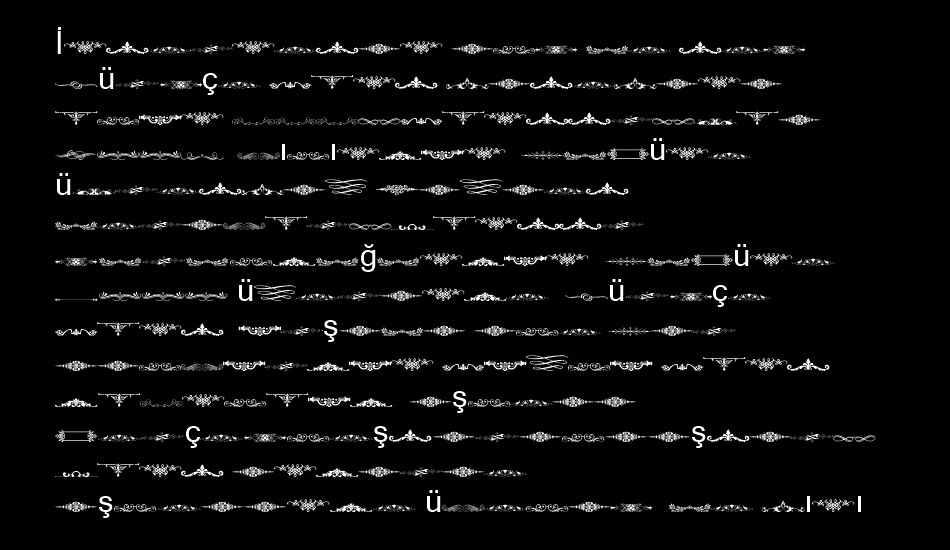The image displays a sequence of text on a solid black background, resembling hieroglyphics but primarily composed of varied and unfamiliar characters, which might suggest an imitation of several writing systems. The text contains a prominent use of certain characters, including the letters 'I' and 'II,' a 'U' with an umlaut (ü), a 'C' with a tail (ç), an 'S' with a tail (ş), and a 'G' with a small crescent on top (ğ).

The topmost line starts with the letter 'I' followed by a series of indecipherable symbols. The second line features the 'Ü' early in the sequence, a 'Ç' mid-line, and more indistinguishable characters following them. The subsequent lines continue in a similar fashion, with various recurring symbols interspersed among continuous enigmatic script. 

From the third to the eighth lines, notable appearances include:
- 'II' and 'Ü'
- 'Ü' separately
- 'Ğ' followed by script
- Repetitive 'Ü' interspersed with other symbols
- A central 'Ş'

This pattern extends through the lower half of the text, where 'Ş' and 'Ç' repeat multiple times, occasionally highlighted by sequences such as 'S tail,' and 'U with the umlaut.' The final lines maintain the character repetition, with scattered symbols, sporadically punctuated by 'II,' creating an overall sense of a structured yet inscrutable script resembling a fusion of various linguistic elements.